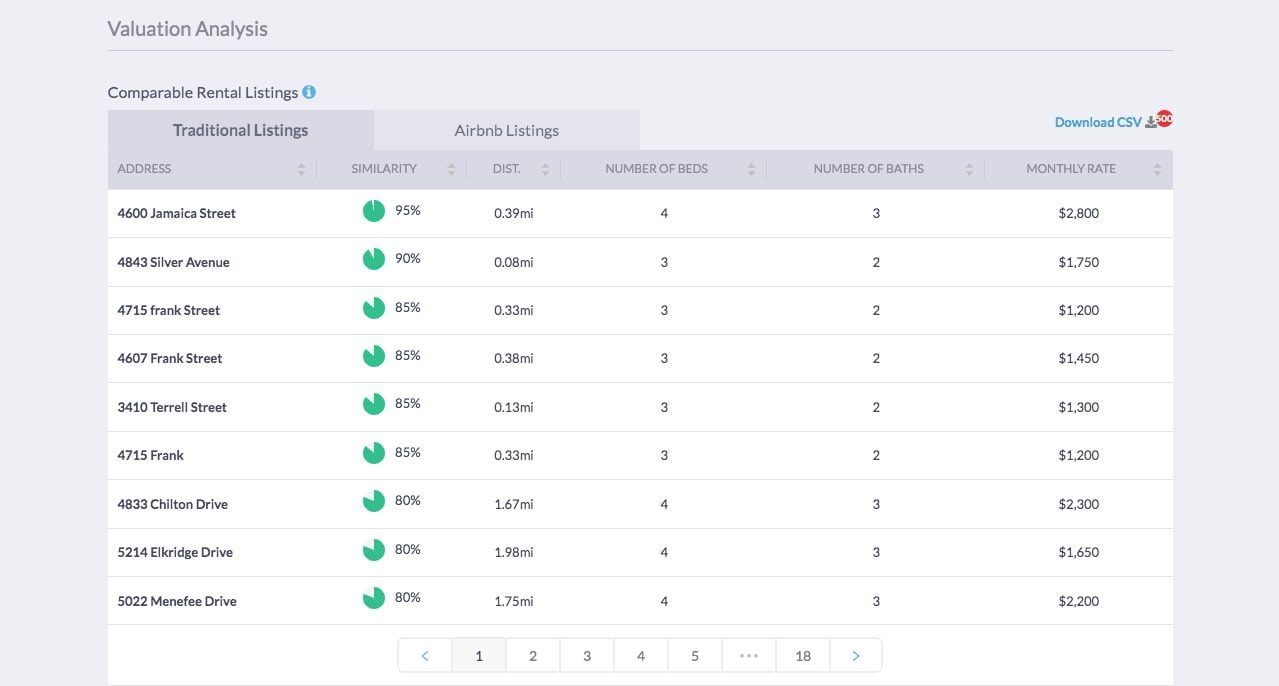This detailed caption describes an image of an analysis tool interface focusing on rental valuations:

---

The image showcases a screenshot of a valuation analysis tool. In the top left corner, the heading "Valuation Analysis" is prominently displayed. Directly below it, the section titled "Comparable Rental Listings" is marked with an information icon enclosed in a blue circle. Two tabs are visible beneath this heading: "Traditional Listings" and "Airbnb Listings," with the "Traditional Listings" tab being actively selected.

A table occupies the main area of the interface, containing columns with headers such as Address, Similarity, Distance, Number of Beds, Number of Baths, and Monthly Rate. The table lists nine entries, each corresponding to different rental properties. Under the Address column, the specific addresses of the properties are listed. The Similarity column features small pie charts indicating the percentage similarity of each property compared to a certain standard or baseline, though the exact comparison criteria are not specified. The Distance column denotes each property’s distance from a fixed location. Number of Beds and Number of Baths columns provide information on the number of bedrooms (either three or four) and bathrooms (either two or three) for each property. The Monthly Rate column lists the rental prices, which range from approximately $1,200 to $2,800.

At the bottom of the table, a pagination control is visible, allowing the user to navigate through multiple pages of listings. It indicates that there are at least 18 pages in total, with the current view displaying page one.

---